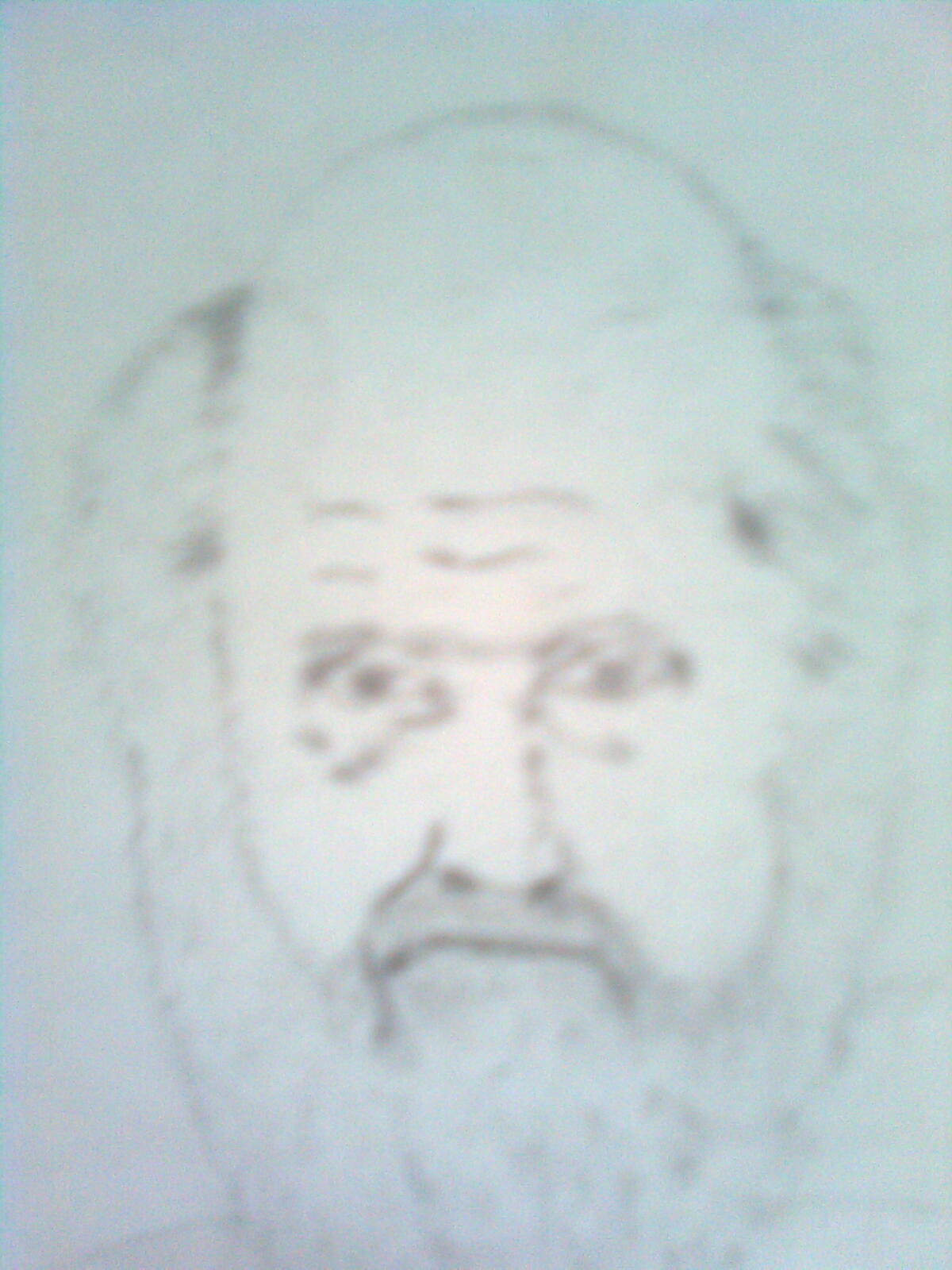This slightly vertical image features a pale bluish-green background that transitions to a lighter, almost white hue near the center. At the heart of this composition is a meticulous charcoal pencil portrait of an older man. The man's hair is sparse on top but dense along the sides of his head, seamlessly blending into a thick, mid-length beard and mustache. His visage is one of solemn contemplation, with deep, dark eyes that gaze directly at the viewer, framed by a wrinkled brow and noticeable bags underneath. The corners of his mouth droop subtly, enhancing the portrait's expression of somber reflection. The artist’s use of charcoal delivers a textured, lifelike quality, emphasizing the character and depth of the gentleman’s features.